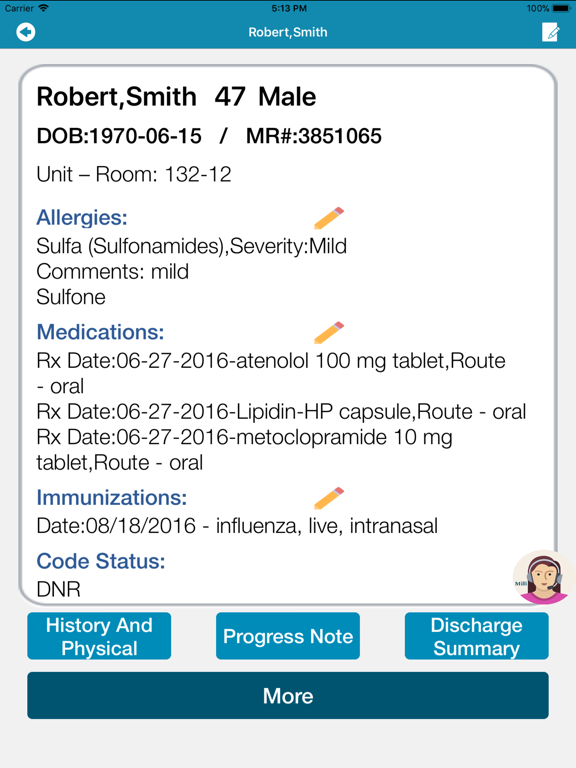Screenshot of a Digital Medical Record on a Smartphone

Captured at 5:13 PM with full Wi-Fi connectivity and a 100% battery charge, this screenshot appears to be from a medical application or website viewed on a smartphone. At the center of the screen, the patient's details are prominently displayed within a white box:

- **Name:** Robert Smith
- **Age:** 47
- **Gender:** Male
- **Date of Birth:** June 15, 1970
- **MR Number:** Not specified (referred to, but details obscured)
- **Unit/Room:** 132-12

In bold blue text, "Allergies" is listed, followed by "sulfa" in black text, with severity and comments both noted as "mild."

Additional sections outline:
- **Medication:** Various tablets and capsules with specific details not provided in this snippet.
- **Immunizations:** A record of the patient's latest immunizations.
- **Code Status:** DNR (Do Not Resuscitate)

At the bottom-right corner of this information box, there is a circular image featuring a cartoon face of a woman with a headset, suggesting a feature for digital or telehealth services. Below this image are three blue tabs lined up horizontally:
1. **History and Physical**
2. **Progress Note**
3. **Discharge Summary**

Finally, a dark blue button spans the entire width of the screen at the bottom, labeled **"More,"** indicating an option to access further details.

Overall, the screen capture depicts a comprehensive digital medical record interface used for patient management, highlighting ease of access to essential medical information and digital health services.